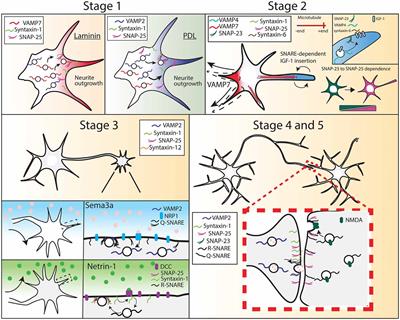The illustration depicts an educational overview of a biological process, shown in multiple stages across several panels. Starting from the upper left and moving left to right, then top to bottom, the image is divided into five stages: Stage 1, Stage 2, Stage 3, with Stages 4 and 5 combined. Each stage demonstrates the progression and changes in cellular structures resembling star-like blobs or cells with arm-like extensions.

In the first panel, labeled "Laminin," and the second, labeled "PDL," the initial forms of the cells are shown. As the stages progress, particularly in Stage 3, the cells exhibit the growth of these arm-like extensions. In the combined Stages 4 and 5, the depiction shows the multiplication of these cells, with secondary formations budding off from the primary shapes, and features moving between different parts of the cells. 

Throughout the illustration, the cells and their components are color-coded in pastel shades of blue, red, purple, and green. Annotations indicate specific proteins and molecules involved at each stage, such as "VAMP7," "Syntaxin1," "SNAP25," "Syntaxin12," "Sema3A," "Netrin-1," and others. These detailed labels point towards the involvement of various SNARE and IGF-1 dependent pathways, indicating a complex sequence of molecular interactions during the cellular processes.